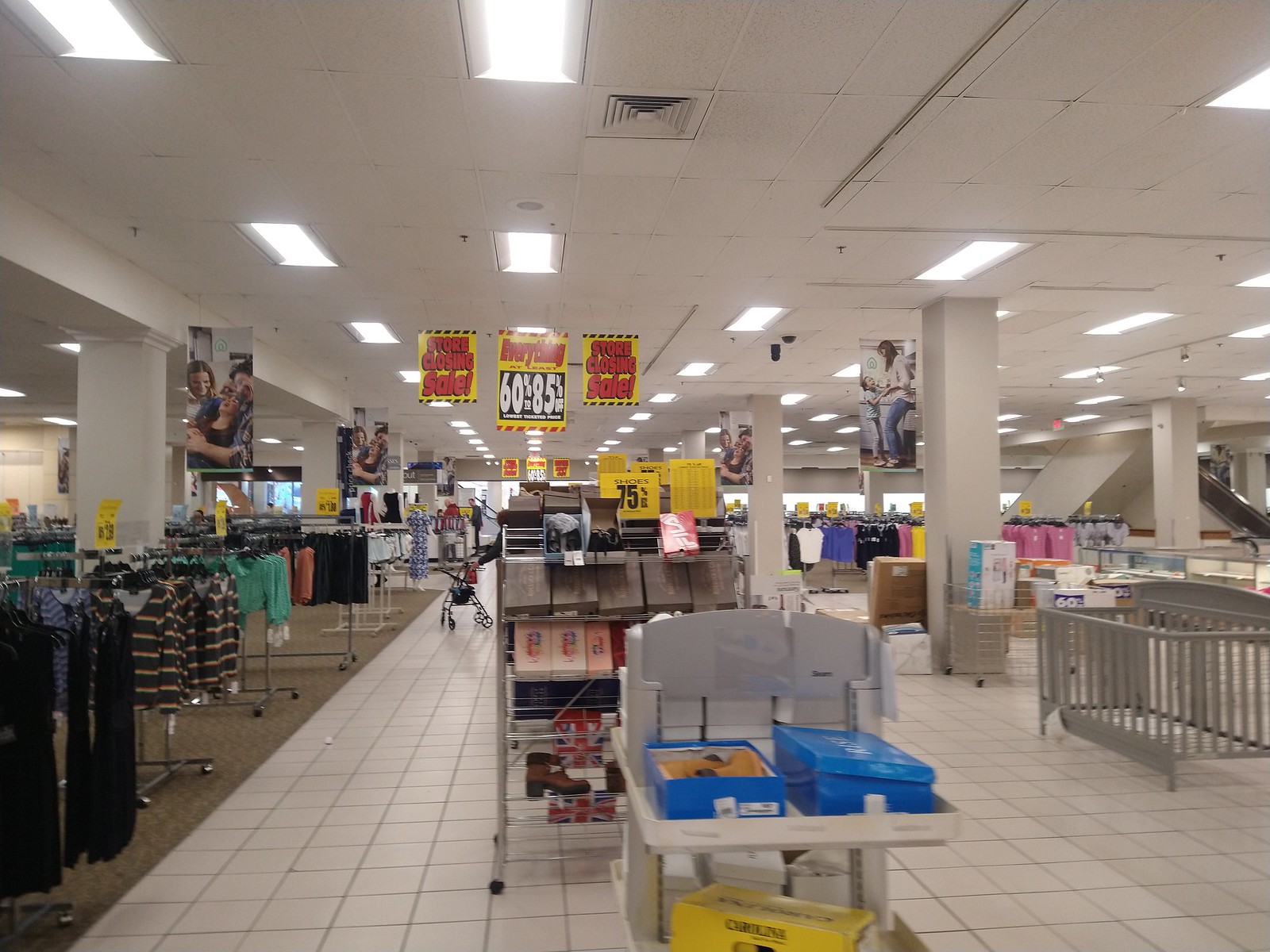This photograph captures the interior of a department store or shopping mall, characterized by its minimalist design. The store features white ceilings and pristine white tile flooring, with plain white columns supporting the structure. There is a noticeable lack of decorative elements, contributing to its stark and utilitarian appearance. In the background, several prominent banners hang from the ceiling, drawing attention with their bold messages. The left and right banners both announce a "Store Closing Sale," while the central banner accentuates the urgency of the event with "Everything at Least 60-85% Off." The store floor is populated with various displays showcasing different items: a baby crib situated on the right side, a mid-section filled with shoe displays, and racks on the left holding assorted clothing such as shirts, pants, and skirts. The overall scene conveys a sense of finality and clearance, highlighting the significant discounts available before the store's impending closure.